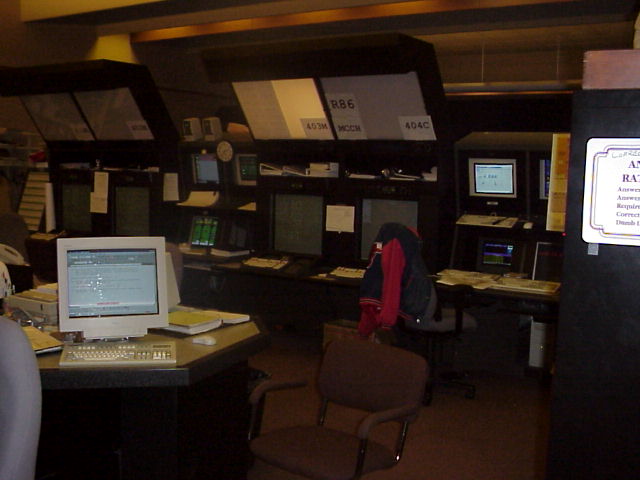The image portrays a dimly lit, vintage-style office or computer lab with a distinctly darker ambiance, accentuated by yellowish lighting. The indoor area lacks windows and features a slightly slanted roof. The left side of the room houses a large, retro white monitor with a matching keyboard positioned on a hexagon-shaped desk. The screen displays indistinct content. The room's carpet is brown, adding to the antiquated feel.

On the right side, a long desk runs the length of the wall, cluttered with various notes and papers. A black and red sweater drapes over the back of a chair. Multiple computer stations dot the room, comprising both desktop computers and smaller, elevated screens. Each station is marked with alphanumeric labels like "45 3N," "R86," "MCCM," and "44C."

Notably, the area is devoid of people. One of the monitors on the right side, perched on a shelf, shows partially visible text that reads "answer require correct something." The overall atmosphere exudes a sense of vintage technology and a workspace frozen in time.